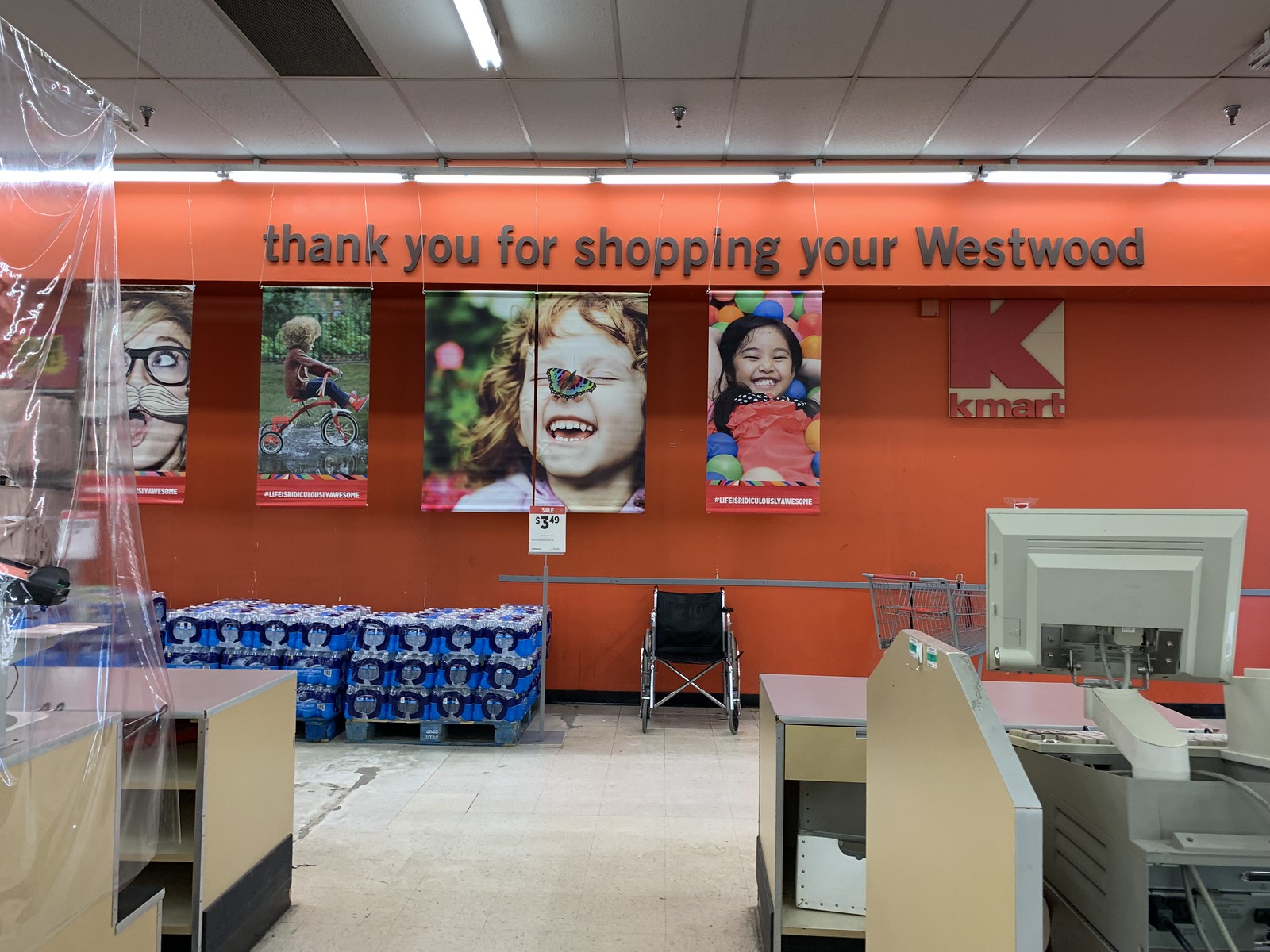A vibrant and bustling interior view of a Kmart store, captured in a photograph. Dominating the right side of the image, a prominent Kmart logo stands out. Moving left from the logo, the store's colorful and inviting decor is highlighted by three vivid photographs of joyful children. The first image showcases a beaming child in a sea of multicolored balls - blues, greens, oranges, and reds - clearly reveling in the playful chaos. The middle photograph features a red-haired girl, a butterfly delicately perched on her nose, her face lit up with laughter. In the third image, another child, possibly a little boy or girl, rides a tricycle gleefully outdoors, undeterred by the rainy weather. Adjacent to these cheerful pictures is a quirky snapshot of a woman with black-rimmed glasses, her face caught in a humorous expression.

Below this lively mural, an assortment of water bottles is strewn across what appears to be a display area, surrounded by various pieces of tan-colored furniture arranged invitingly. The background is punctuated by an orange wall with a thank you message for shoppers, reading "Thank you for Shopping. You're a Westwood." Beneath this message, the familiar Kmart logo reappears, reinforcing the store's brand and welcoming customers.